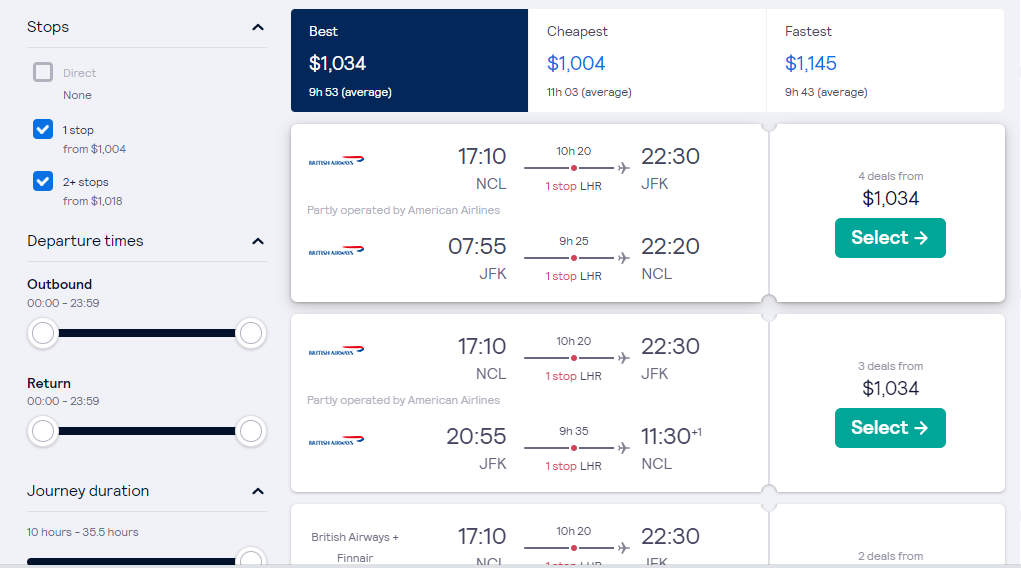**Detailed Caption:**

This screenshot, taken from an unidentified travel website, showcases a section of the flight search results page. On the left-hand side, there's a vertical menu dedicated to filtering options for stops. The options include: "Stops" with sub-options "Direct (None)," which is unchecked, "One Stop for $1,004," which is checked, and "Two Plus Stops for $1,018," also checked. Additionally, filters for "Departure times" indicate outbound and return journeys available from 00:00 to 23:59. "Journey duration" options range from 10 hours to 35.5 hours.

On the right side, a detailed breakdown of flight costs and durations is visible. The "Best" option is priced at $1,034, with an average duration of 9 hours and 53 minutes. The "Cheapest" flight costs $1,004, averaging 11 hours and 3 minutes. The "Fastest" flight is priced at $1,145 and takes approximately 9 hours and 43 minutes on average.

Below this, specific flight details are provided:
- **First flight option:** Operated by British Airways in collaboration with American Airlines, departing from NCL at 17:10, with a duration of 10 hours and 20 minutes, making a stop at LHR, and arriving at JFK at 22:30. The return leg departs JFK at 07:55, with a duration of 9 hours and 25 minutes, including a stop at LHR, and arrives at NCL at 22:20. This option offers four deals priced at $1,034, available for selection.
  
- **Second flight option:** Also operated partially by British Airways and American Airlines, departing from NCL at 17:10, with a duration of 10 hours and 20 minutes, stopping at LHR, and arriving at JFK at 22:30. The return flight departs from JFK at 20:55, lasting 9 hours and 35 minutes, with a stop at LHR, and arrives at NCL at 11:30 the next day. This option offers three deals priced at $1,034, available for selection.
  
- **Third flight option:** Operated by British Airways in combination with Finnair, departs from NCL at 17:10, with a 10 hour and 20 minute trip arriving at JFK at 22:30. The remaining details of this option are cut off due to the lower edge of the image.

The layout and filtering options suggest a user-friendly approach to finding the most suitable flights based on price, duration, and number of stops.